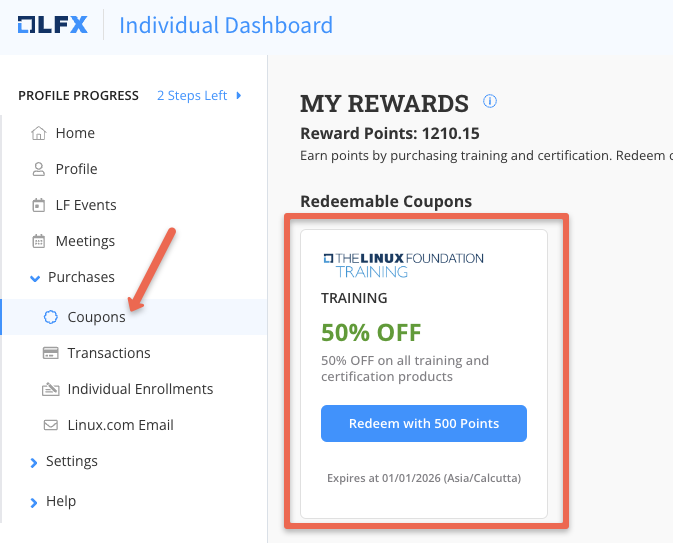The image depicts a website named "OLFX," featuring its name prominently in blue and black letters. At the top of the page, a navigation bar labeled "Individual Dashboard" displays sections such as "Home," "Profile," "LF Events," "Meetings," and "Purchases." Each section comes with a drop-down arrow for further options. Additionally, the navigation bar includes a notification in white text stating “Profile Progress: Two Steps Left.”

Beneath this bar, there are several options such as "Coupons" marked with a long red arrow highlighting the section. Following this are sections for "Transactions," "Individual Enrollments," "Links.com," "Email Settings," and "Help."

On the right-hand side of the website, a "My Rewards" section is visible, displaying the following details: "Reward Points: 1210.15" and a message encouraging users to "Earn points by purchasing training and certification." It also features a partially displayed "Redeem" button before being cut off.

The "Redeemable Coupons" section contains a red-outlined box housing a white box inside. Within this, it shows an offer from "The Limnox Foundation Training," detailing a green-highlighted “50% off” discount message for all training and certification products. Below this, a blue bar states, "Redeem with 500 points," and includes an expiration note: "Expires on 01/01/2026, Asia/Calcutta."

This detailed layout provides comprehensive navigation and reward details focusing on user engagement through training and certification benefits.